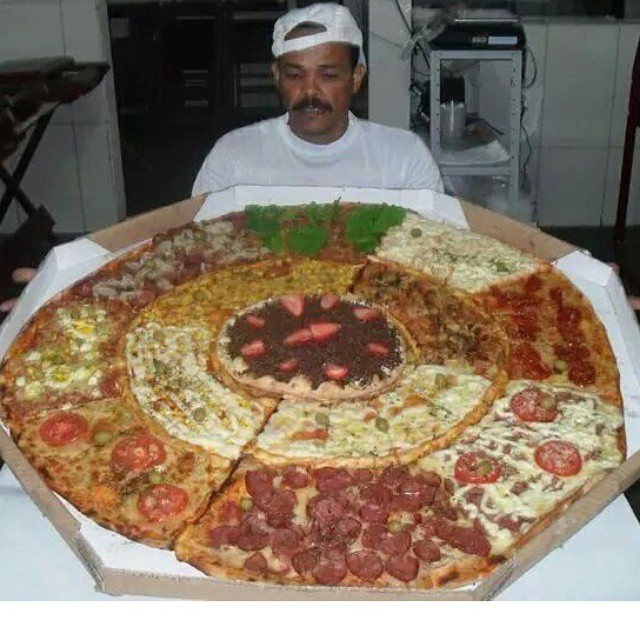This image showcases an enormous, meticulously sectioned pizza, likely around three feet in diameter, set on a cardboard holder. Each segment of this colossal pizza boasts unique toppings, highlighting a diverse array of flavors and colors. Starting from the bottom, there is a pepperoni section encircling the edge. Adjacent sections feature tomatoes paired with green herbs, a colorful mix of red, yellow, and green ingredients, followed by sections with brown and red toppings, one with fresh green leaves, and a predominantly yellowish-white area accented with green. There's also a segment with a reddish-brown and light brown combination, and another showcasing tomatoes, greens, and cheese. The central intersections of the pizza display a consistent yellow-green hue with a few red spots, an orangey-brown section to the left, blending into browns and reds to the right, and one striking area that appears chocolatey-brown with strawberries.

A man stands behind the pizza, gazing down at it. He has a mustache, short hair, and wears a backwards white baseball cap along with a white t-shirt. His darker skin tone contrasts with his clothing. The pizza, dwarfing the man's shoulders, occupies the bottom to the middle of the image, emphasizing its massive size, seemingly about double the width of the man's shoulders and consuming about 60% of the visual space. The indoor setting adds to the focus on the pizza and the man's curious expression.